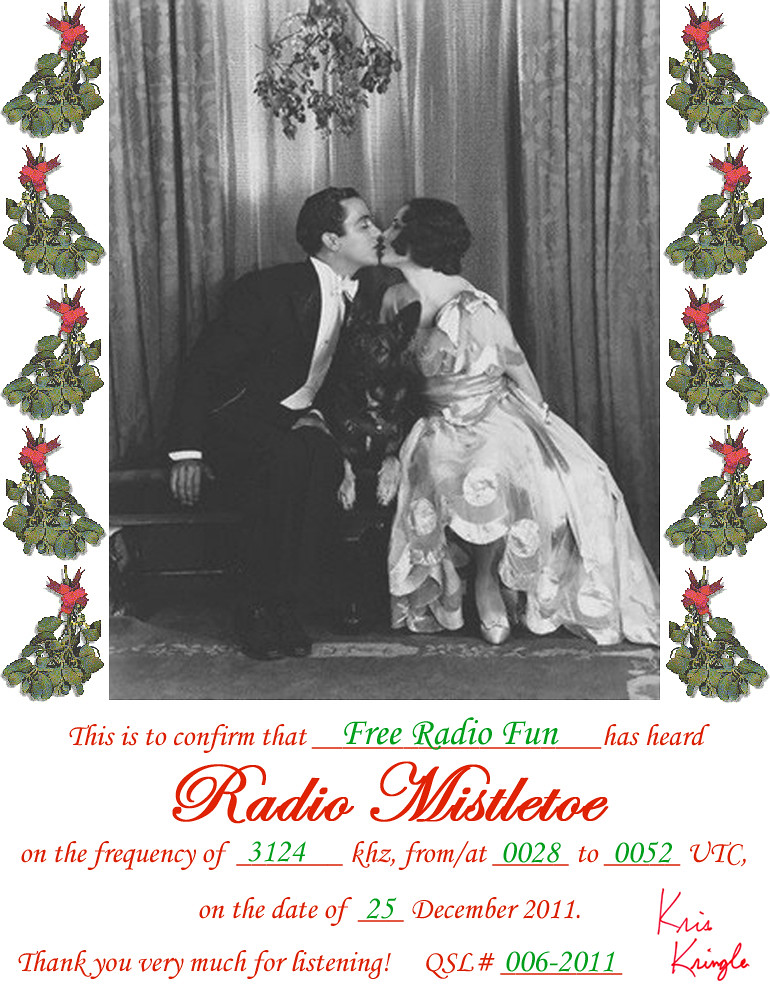This image, reminiscent of a vintage postcard, captures a black and white photograph from what appears to be the 1930s. Centrally displayed is a couple about to kiss under a sprig of mistletoe, framed by lush curtains. The man, donned in a tuxedo with a white bow tie, and the woman, elegantly dressed in a full-length gown, exude timeless romance. Seated intimately close, a German Shepherd dog sits obediently between them. Surrounding this nostalgic scene, rows of mistletoe, each tied with a red ribbon, add a festive touch. Below, in festively colored text, it reads: "This is to confirm that Free Radio Fun has heard Radio Mistletoe on the frequency of 3124 kHz from 0028 to 0052 UTC on the date of 25th December, 2011. Thank you very much for listening. QSL number 006-2011." The message is signed in red cursive as "Kris Kringle," adding a final holiday flourish.